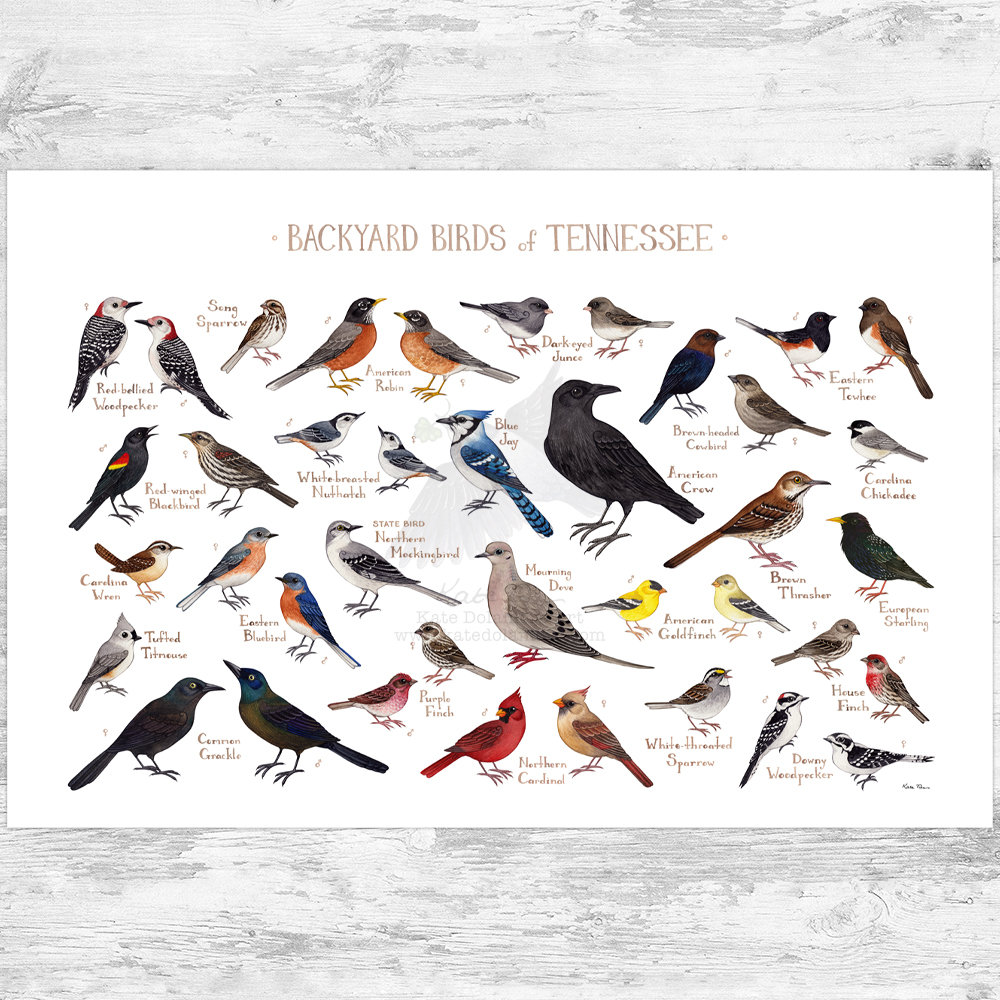The image depicts a detailed, stylized drawing reminiscent of the Audubon bird book, titled "Backyard Birds of Tennessee" in grayish writing against a white background. This poster showcases a vibrant array of approximately 25 to 50 birds, each identified by name. Among the identifiable species are the American robin, blue jay, northern cardinal, red-winged blackbird, eastern bluebird, tufted titmouse, red-bellied woodpecker, white-breasted nuthatch, American goldfinch, white-throated sparrow, Canadian wren, song sparrow, and downy woodpecker. The birds are illustrated in their natural hues—reds, blues, yellows, oranges, and blacks—adding a colorful and informative element to the wooden wall or table backdrop on which this poster is displayed.